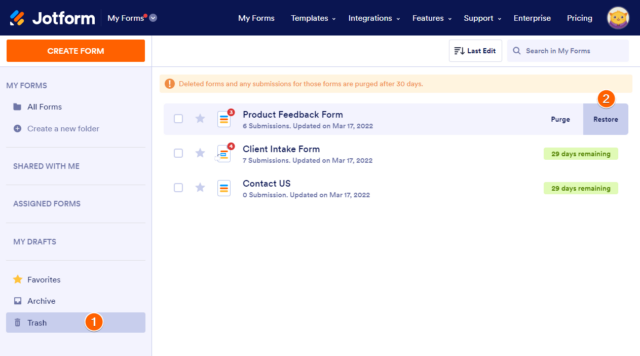The image is a screenshot from the JotForm website. At the top of the page, there is a blue navigation bar. On the left side of the bar, next to the word "JotForm," there is a logo consisting of blue, red, and yellow elements. To the right of the logo, the navigation bar includes the options: "My Forms" with a dropdown menu, "Templates," "Integrations," "Features," "Support," "Enterprise," and "Pricing."

Below the navigation bar, on the left side, there is a prominent "Create Form" button. Under this button, a vertical sidebar lists several sections: "My Forms," "Shared With Me," "Assigned Forms," "My Drafts," "Favorites," "Archive," and "Trash."

In the main content area to the right, there is a white box containing sections for various form types, such as "Product Feedback Form," "Client Intake Form," and "Contact Us Form." At the top right corner of this section, there is an option labeled "Last Edit" and a search box. Additionally, there is an image of what appears to be a hamster or mouse included on the page.

This detailed layout captures the structured interface and diverse options available to users on the JotForm website.